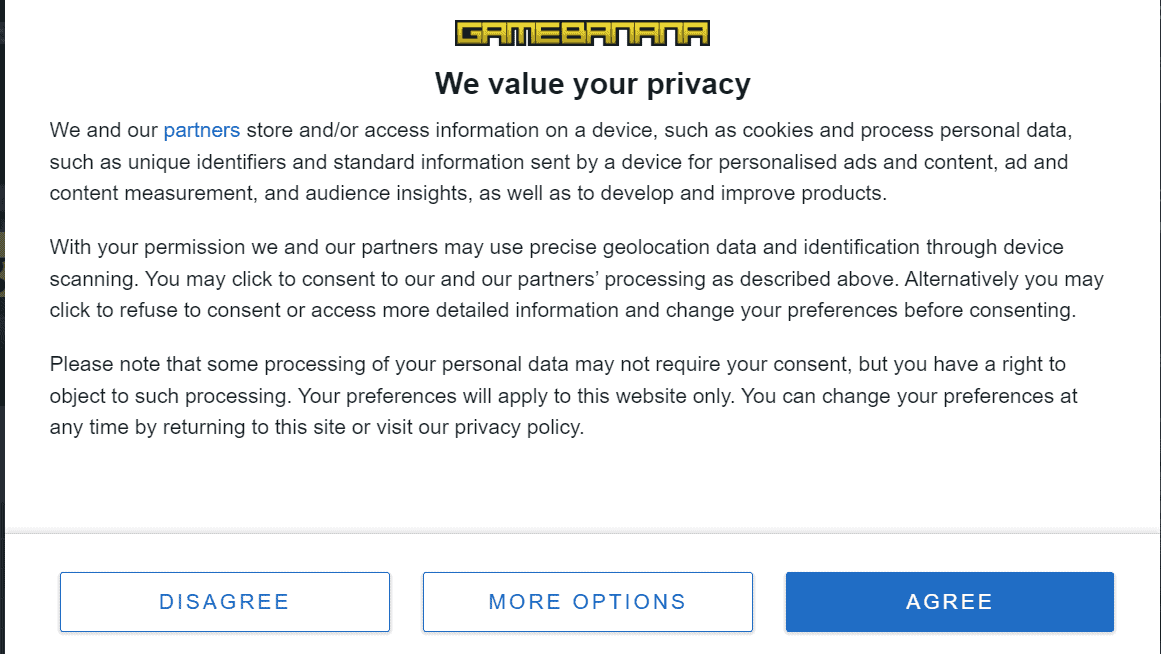**Caption:**

The screenshot captures a desktop notification with a predominantly white background. At the top center of the image, bold yellow text displays "GameBanana" as a single word. Directly beneath this header, the text "We value your privacy" is prominently shown.

The notification elaborates in a detailed description: "We and our partners" (with "partners" hyperlinked in blue) store and/or access information on a device, using cookies to process personal data. This includes unique identifiers and standard information sent by a device for personalized ads and content, ad and content measurement, audience insights, and to develop and improve products. It specifies that, with user permission, precise geolocation data and identification through device scanning may be used. 

Users are given options to consent to these processes or access more detailed information to manage preferences before consenting. The text clearly states that some processing of personal data might not require consent, but users have the right to object to such processing. Preferences can be changed at any time by returning to the site or visiting the privacy policy.

At the bottom of the screenshot, three rectangular buttons are displayed: "Disagree," "More Options," and a blue "Agree" button.